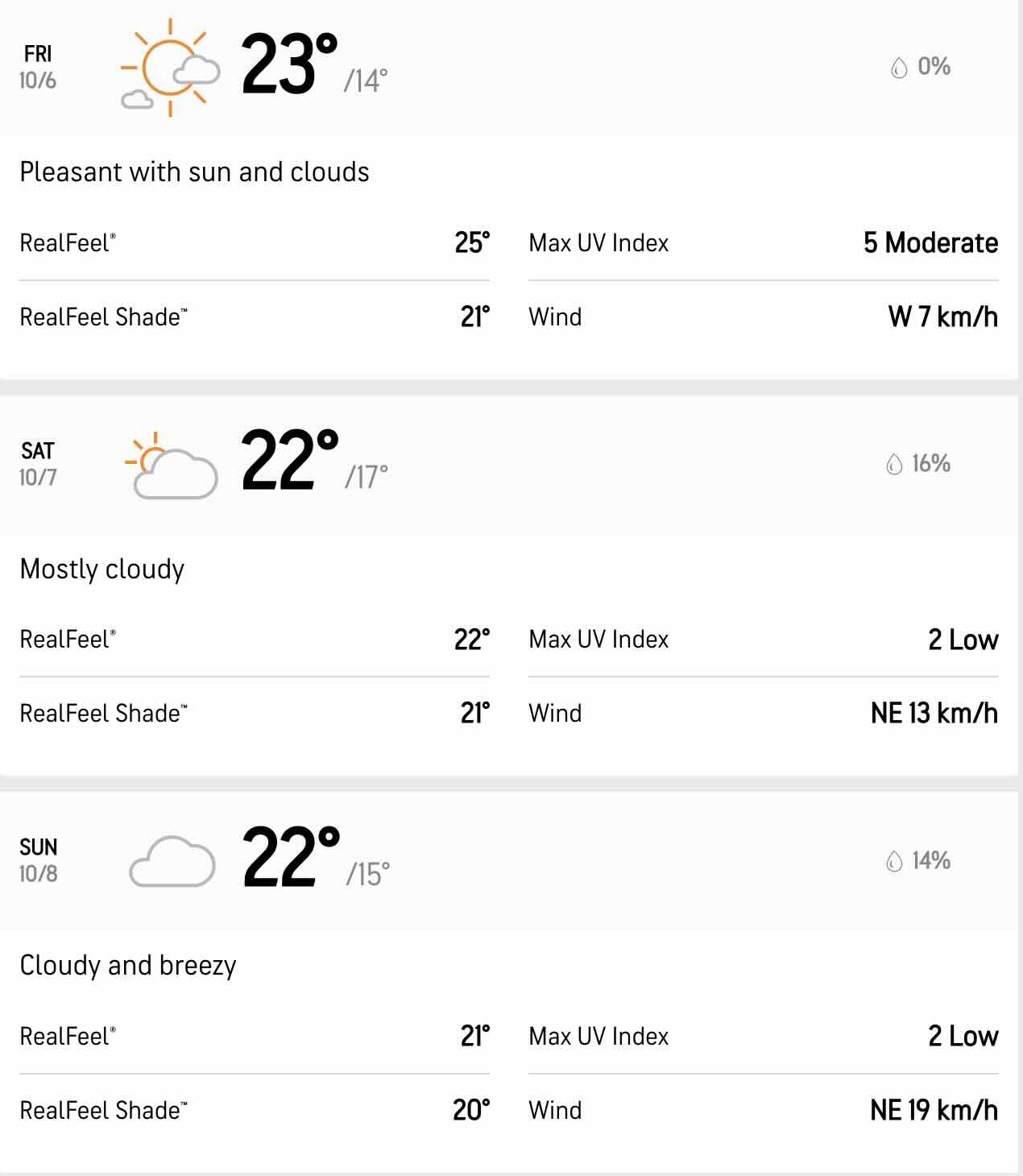### Detailed Weather Forecast for the Weekend

**Friday, October 6:**
- **Conditions:** Pleasant with sun and clouds
- **Temperature:** 23°C (14°F)
- **Real Feel:** 25°C (77°F)
- **Real Feel in Shade:** 21°C (70°F)
- **Precipitation:** 0%
- **UV Index:** 5 (Moderate)
- **Wind:** West at 7 km/h

**Saturday, October 7:**
- **Conditions:** Mostly cloudy
- **Temperature:** 22°C (72°F) with a low of 17°C (63°F)
- **Real Feel:** 22°C (72°F)
- **Real Feel in Shade:** 21°C (70°F)
- **Precipitation:** 16%
- **UV Index:** 2 (Low)
- **Wind:** Northeast at 13 km/h

**Sunday, October 8:**
- **Conditions:** Cloudy and breezy
- **Temperature:** 22°C (72°F) with a low of 15°C (59°F)
- **Real Feel:** 21°C (70°F)
- **Real Feel in Shade:** 20°C (68°F)
- **Precipitation:** 14%
- **UV Index:** 2 (Low)
- **Wind:** Northeast at 19 km/h

*This image is a screenshot from a weather overview website, providing a detailed and organized summary for the upcoming three days: Friday, Saturday, and Sunday.*